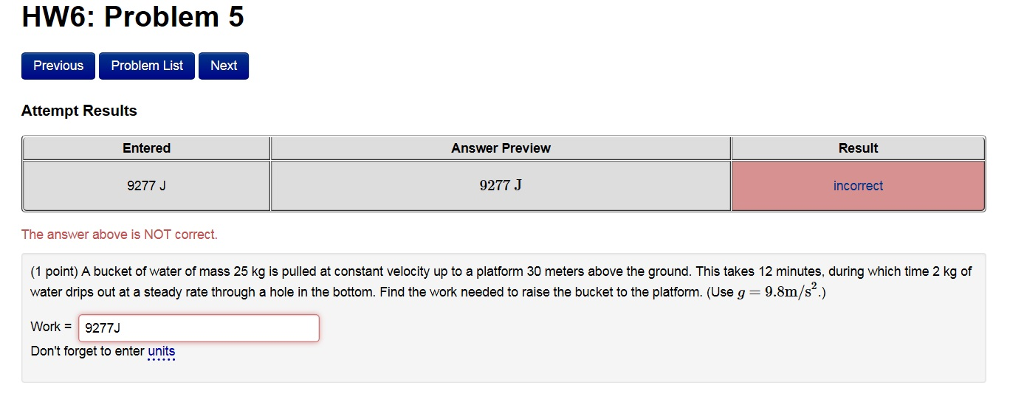Title: HW6: Problem 5 - Learning Tool Interface

The learning tool interface for HW6: Problem 5 is displayed prominently at the top. Below the title, there are three blue buttons with white text: "Previous" on the left, "Problem List" in the center, and "Next" on the right.

Underneath these navigation buttons, there is a section labeled "Attempt Results" which features a chart. The chart includes headers and one row of data displaying:
- Entered: 9277J
- Answer Preview: 9277J
- Result: Incorrect

Despite the matching entries in the "Entered" and "Answer Preview" columns, it indicates that the answer is incorrect. Directly below, a message confirms, "The answer above is not correct." 

The problem statement is then presented:
"A bucket of water of mass 25 kilograms is pulled at a constant velocity up to a platform 30 meters above the ground. It takes 12 minutes, during which time 2 kilograms of water drip out at a steady rate through a hole in the bottom. Find the work needed to raise the bucket to the platform. Choose \( g = 9.8 \, \text{m/s}^2 \)."

At the bottom of the interface, there is a red-outlined box where the attempted answer, "Work = 9277J", is displayed. A reminder in blue text prompts: "Don't forget to enter units."